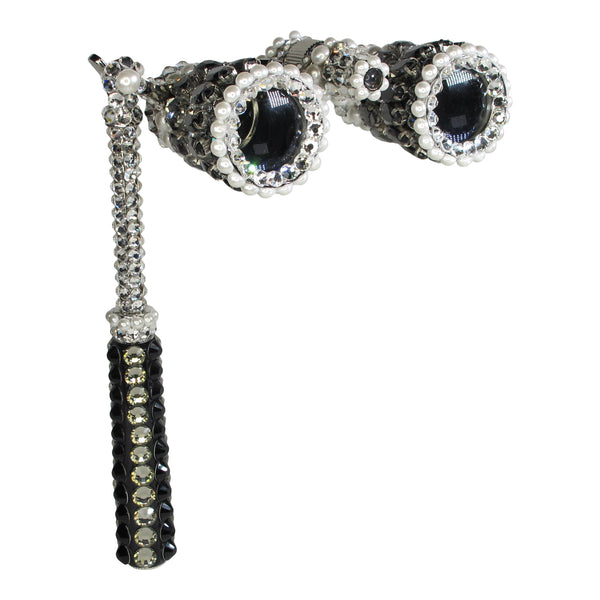The image depicts an ornate pair of opera binoculars, mounted on a handle-like rod for easy use with the right hand. Unlike typical bird-watching binoculars, these are designed for use in a theater or opera house to view performers from a distance. The entire device exudes luxury, being lavishly encrusted with a combination of white pearls and glittering silver stones, which may be rhinestones, creating a striking, classy appearance. The handle, predominantly black, is also detailed with silver stones, adding to the opulent design. The lenses are notably very black, contrasting sharply with the sparkling embellishments and reflecting light elegantly. The background of the image is a pristine white, further highlighting the exquisite and gaudy craftsmanship of the binoculars. Additionally, a reflection in the glass lenses might even reveal an American flag.